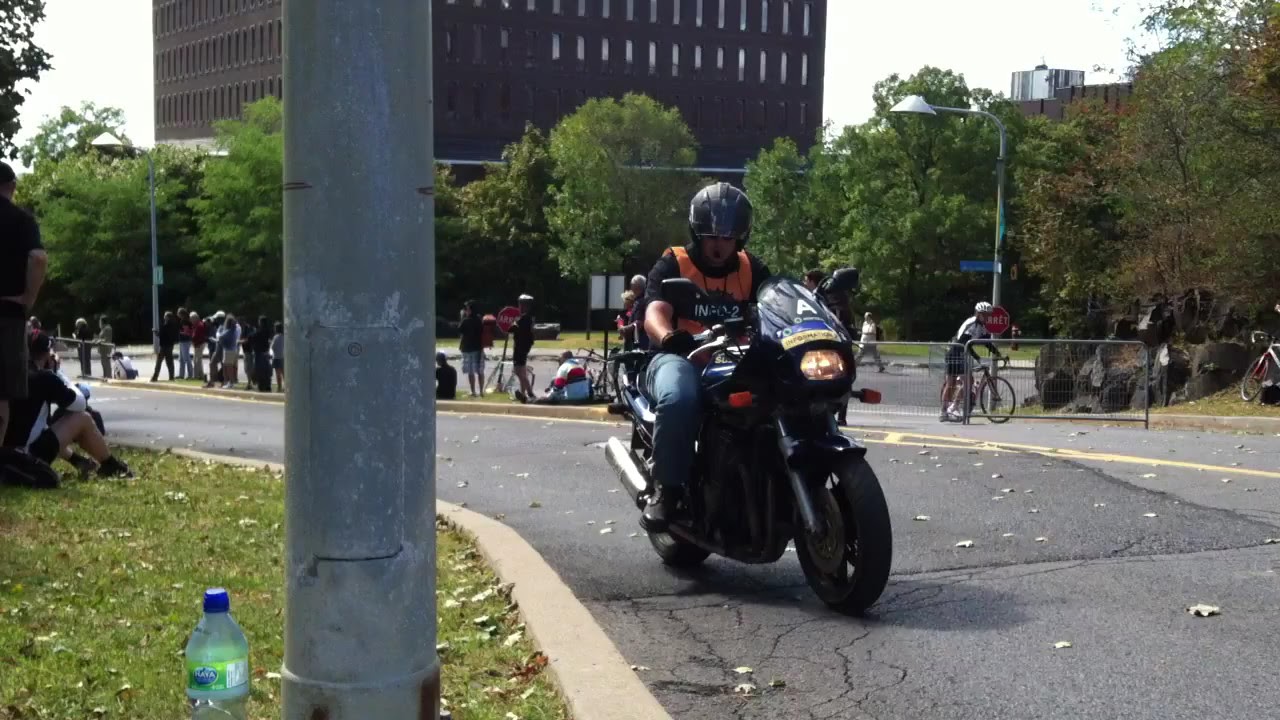In this detailed city scene, the central figure is a man riding a motorcycle, which is coming up from the center of the image towards the viewer. He is wearing a black helmet, a black t-shirt, a distinct orange safety vest, and blue jeans. The motorcycle has a front yellow light turned on and a small windshield emblazoned with the letter "A." The road he rides on is slightly curved and flanked by patches of grass.

In the bottom left corner of the image, a patch of grass contains a gray streetlamp pole, next to which sits a bottle of water with a blue lid and a green label. Nearby, there are two people in dark clothing sitting in the grass, indicating a relaxed, communal atmosphere. To the right of the rider, a bicyclist is seen getting back on his bike.

A large number of people are scattered on the grass median, suggesting a park or college campus setting. This grassy area is lined with trees and backgrounded by a sizable, six-story brick building. The scene is bathed in daylight, with colors ranging from green, blue, gray, and orange, to yellow, red, white, black, and brown, contributing to the lively and detailed outdoor urban snapshot.